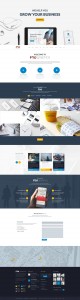A screenshot of a smartphone displaying a very blurry web page. The quality of the image makes it difficult to distinguish specific details clearly. At the top, there appears to be a header resembling the combination of a tablet and a pen, suggesting it might be an iPad or a similar device. Below this header are three blue settings wheels. There are several rows of images, though the content of these images is indiscernible. One image below these appears to show a person holding a smartphone in their left hand. Farther down the page, there are indistinct sections with varying background colors, such as white and gray. No legible text is visible in the screenshot. Overall, the webpage seems to be showcasing a product rather than a service, although the exact nature of the product remains unclear due to the blurriness of the image.